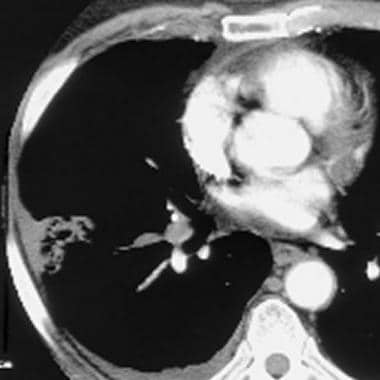This black and white image, likely an x-ray or similar medical scan, showcases a striking contrast between dark and light areas, primarily in a monochrome palette. The background is solid black, emphasizing the white and grey anatomical features present in the foreground. Dominating the center-right portion of the image is a segmented white mass comprised of three sections with greyish edges, giving the appearance of soft tissue or a formation within a bodily structure. Below this mass, slightly to the right, lies a circular white shape bordered by grey, possibly indicating a round anatomical feature or lesion.

Encircling the upper left and lower right corners of the image is a grey-white ring that might resemble the curvature of ribs or a similar skeletal structure. This ring frames the central elements and adds to the complexity of the scan. To the lower left of the primary mass, an irregularly shaped object or collection of objects can be observed, suggesting the presence of various tissues or anatomical components densely packed in this region.

Overall, the image exudes an intricate and slightly enigmatic medical composition, with a black backdrop enhancing the clarity and prominence of the white and grey anatomical details within the square frame.